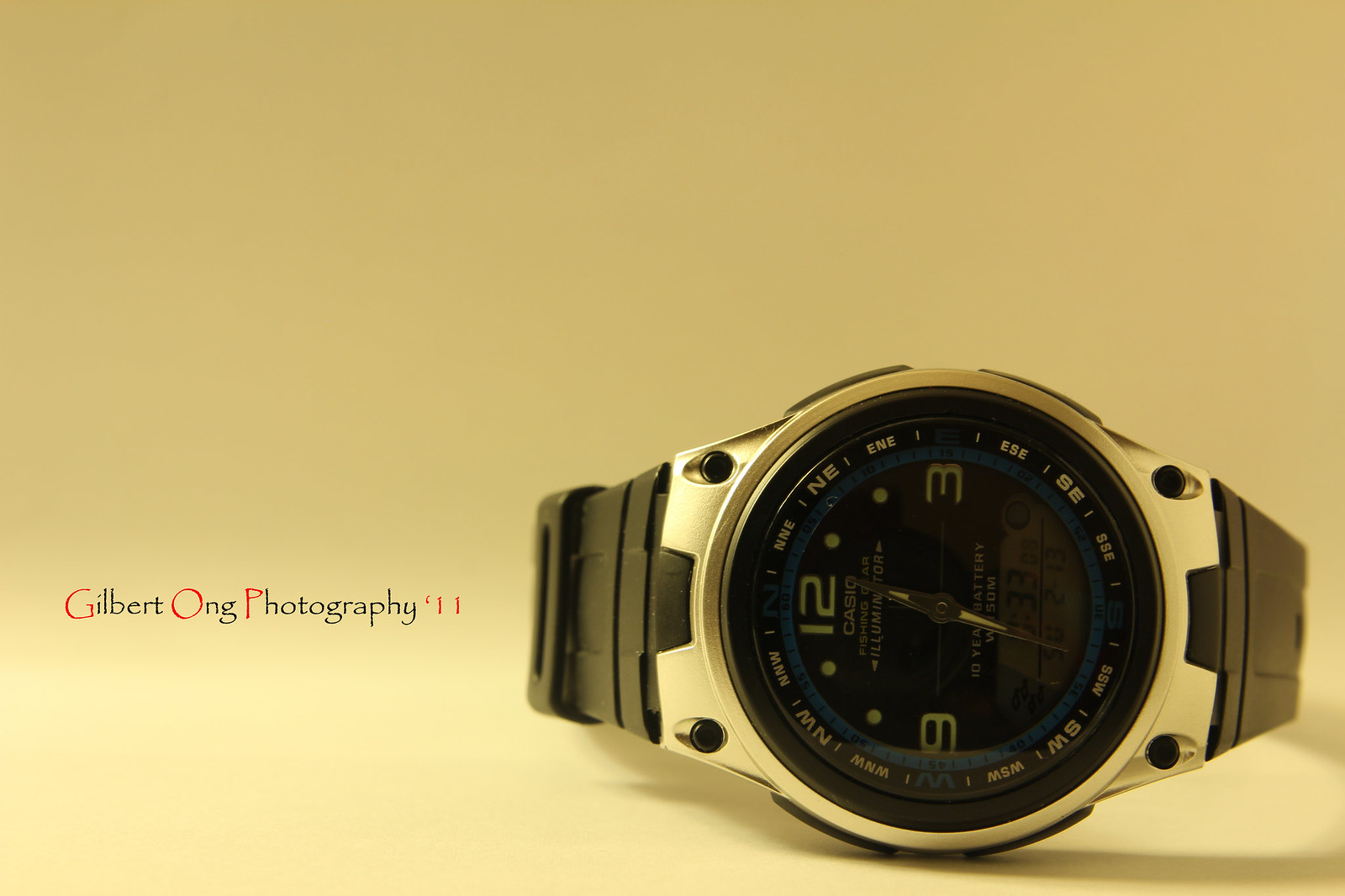This photograph captures a detailed image of a watch against a tan background that lightens towards the bottom, suggesting a reflective surface. On the left side of the image, the text "Gilbert Ong Photography" is printed, with the initials "G," "O," and "P" highlighted in red while the remaining letters are in black. Adjacent to the word "Photography," the number "11" appears in red.

The primary focus of the image is a watch situated to the right. The watch features a round, steel dial and a band that seems to be made of either leather or plastic. The face of the watch is predominantly black with a hint of blue around the dial. The watch includes directional markers, such as northeast and southwest, suggesting it is a navigational timepiece.

The dial is marked with the numbers 12, 3, 6, and 9, though the number 6 is partially obscured at the lower edge.